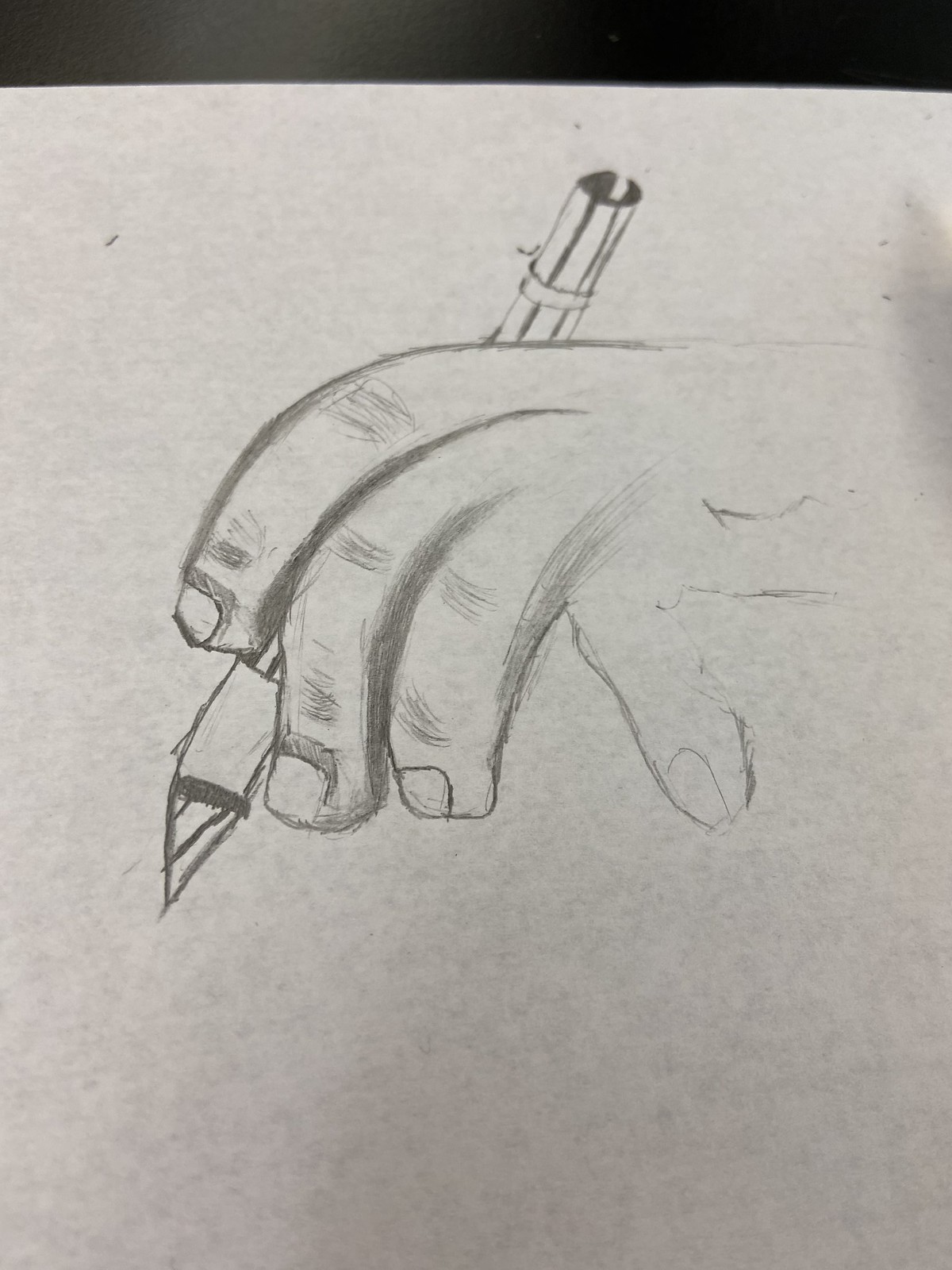This is an intricate pencil drawing rendered on a pristine white sheet of paper, depicting a hand grasping a writing utensil. The utensil held by the hand, which could be a pencil or pen, features a notably pointed, triangular tip—a focal point that emphasizes precision. The artist has elaborately shaded the knuckles, adding depth and texture to the hand, which prominently displays three fingers, while the pinky finger is only faintly visible, emerging at an awkward angle. The hand’s fingertips and nails are distinctly square, adding to the detailed realism of the sketch. The upper end of the pencil or pen is incomplete, notably missing any end cap or eraser, giving it an unfinished appearance. Some line work has been attempted to enhance realism, contributing to the overall intricacy of the drawing.